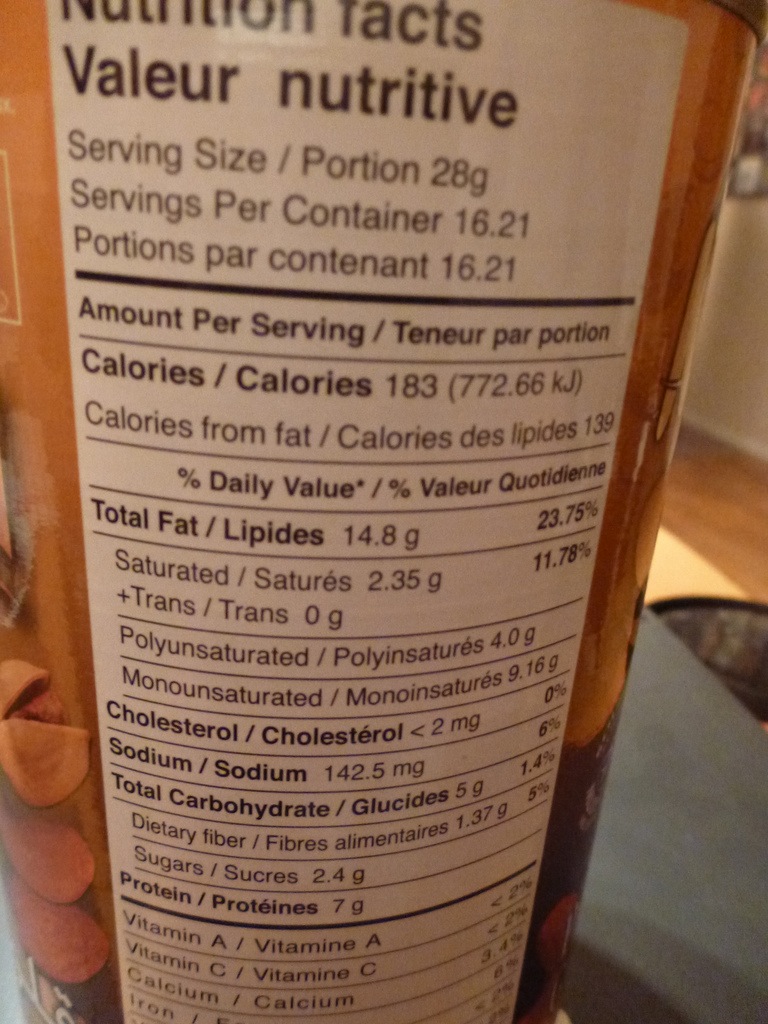A close-up photograph captures a bilingual nutritional label from a product, likely from a region such as Canada where both English and French are commonly used. The label prominently features the headings "Nutrition Facts" and "Valeur Nutritive." It details a serving size of 28 grams with approximately 16.21 servings per container. 

The nutritional information per serving includes:
- Calories: 183
- Total Fat (Lipides): including breakdowns of saturated, polyunsaturated, and unsaturated fats
- Cholesterol: less than 2 milligrams
- Sodium: 142.5 milligrams
- Total Carbohydrates: 5 grams, which includes 1.37 grams of dietary fiber and 2.4 grams of sugar
- Protein: 7 grams

The label also notes negligible amounts of Vitamin A, Vitamin C, calcium, and iron. The lower portion of the label extends off the bottom of the photo, indicating there may be additional information not captured in the image.